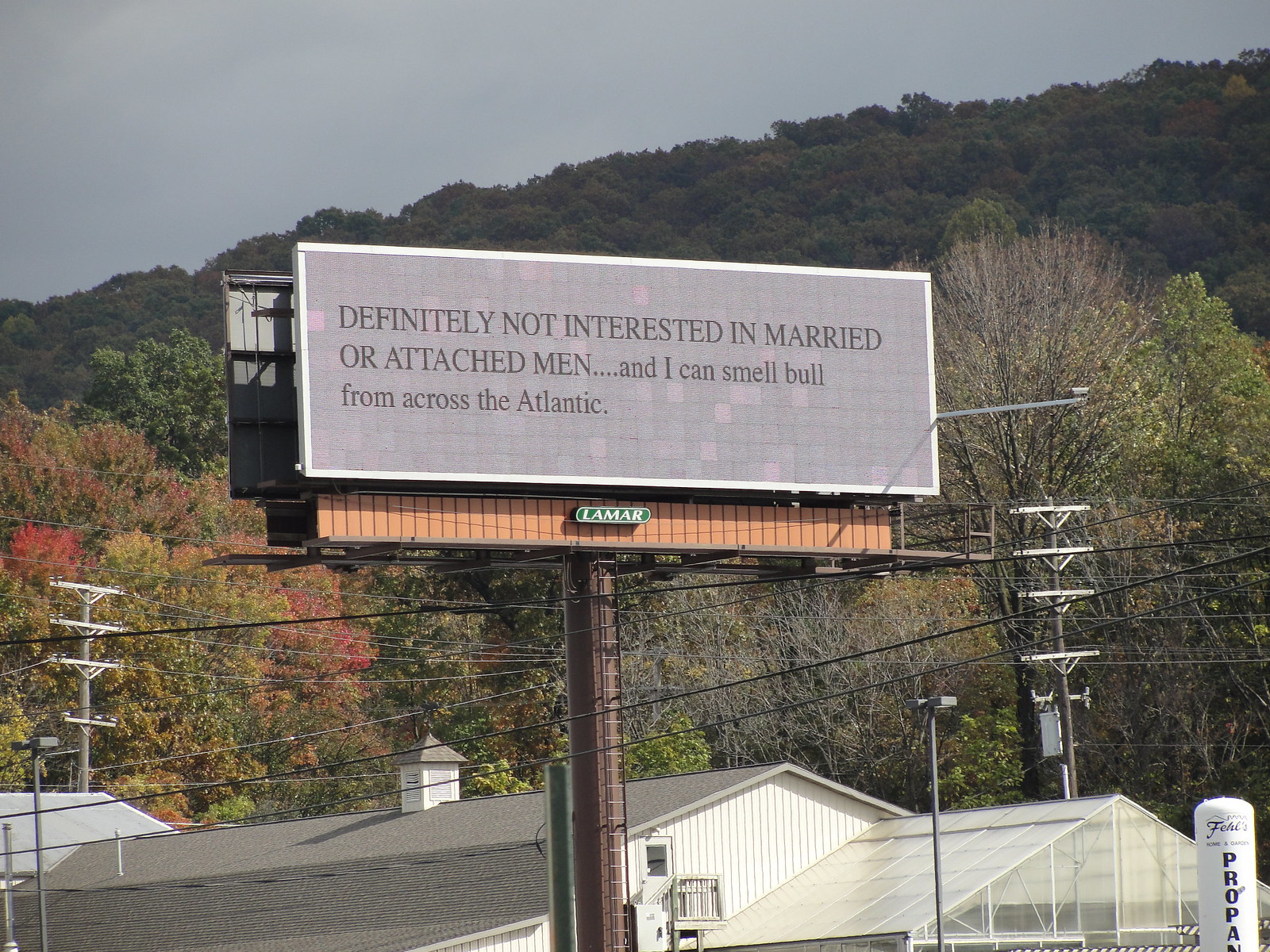The image showcases a serene setting with a pale gray sky as the backdrop, complemented by rolling hills densely covered in trees adorned with a vivid palette of red, green, and yellow autumn leaves. In the foreground, there's a white, elongated propane workshop prominently featuring a large, distinctive sign shaped like a propane tank with black lettering. Nearby, an eye-catching street sign with a gray background and bold black text humorously declares, "Definitely not interested in married or attached men and I can smell bull from across the Atlantic." The scene is interspersed with several light poles and an intricate web of overhead lines, adding a touch of urban complexity to the otherwise natural landscape.